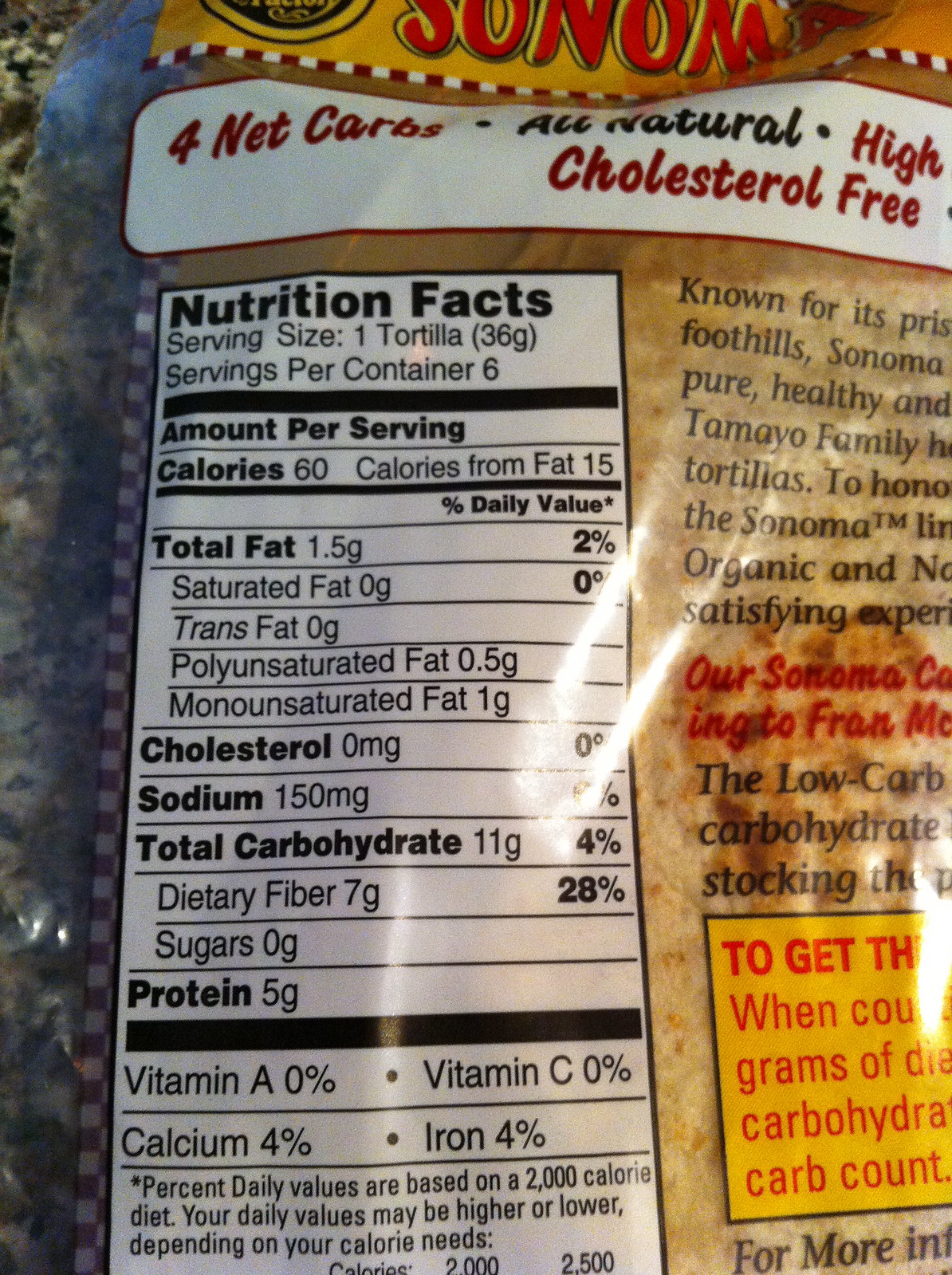This detailed image captures a close-up of the back of a tortilla bag, positioned on a gray and black speckled granite counter. The tortilla is packaged in a clear plastic bag, revealing light brown tortillas inside. The top of the bag prominently features the brand name "Sonoma" in red with a yellow outline, followed by a white banner proclaiming "4 net carbs, all natural, high cholesterol free."

The left side of the image shows the nutritional facts, printed in black on a white background, organized in a detailed chart format. The information includes serving size (one tortilla), servings per container (six), and various nutritional details: 60 calories per serving with 15 calories from fat, 1.5 grams of total fat (2% daily value), 0 grams of saturated fat, trans fat, polyunsaturated fat, and monosaturated fat. Additionally, it lists 0 milligrams of cholesterol and 11 grams of total carbohydrates.

To the right of the nutritional chart, there's text providing more information about the bread, though it's cut off and partially visible. The text is written in black font, with a red section reading "Our Sonoma" and additional details presented in a yellow and red area towards the bottom. This red and yellow section seems to contain more product information.